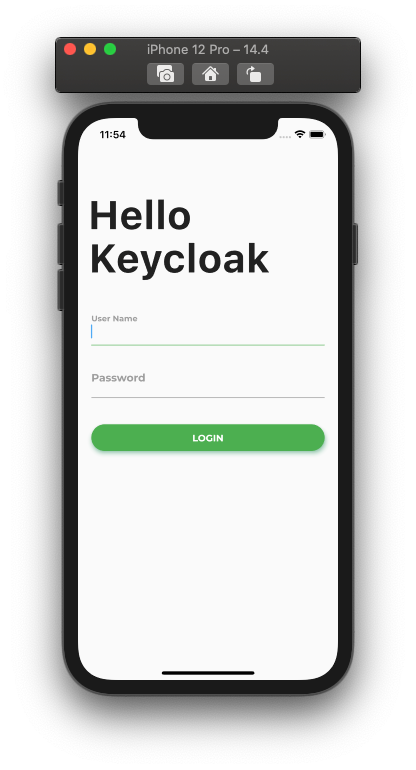This vertical image displays a screenshot of an iPhone 12 Pro with iOS version 14.4. The entire black phone is shown, framed by a misty grey shadow. Above the phone, a dark grey floating header features three colored dots—red, yellow, and green—positioned at the upper left-hand corner. Centered beneath the label “iPhone 12 Pro-14.4” are three icons on grey backgrounds: a white camera, a white house, and a white square with a right-facing curved arrow.

The phone's screen shows the time as 11:54 in the upper left-hand corner, with a status bar and battery indicator on the upper right. Dominating the screen in large black text are the words "Hello Key Cloak." Below, there is a field labeled “username” in small grey text, accompanied by a vertical thin blue bar; the username field is empty. A thin green horizontal line highlights the area beneath this section. Following this is a larger "password" field, also in grey text, above a thin grey horizontal line. At the bottom of the screen, a wide green button with "LOGIN" in white capital letters stands out, along with a short black horizontal line at the bottom edge of the phone's screen.